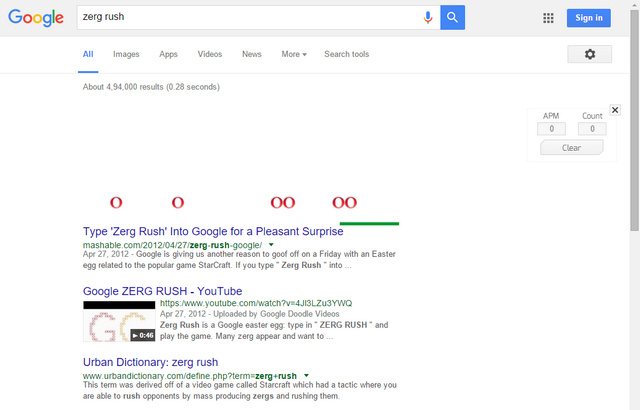This detailed caption describes a screenshot of a Google search page:

The image depicts a screenshot of a web version of a Google search results page. At the very top, a gray navigation bar features the colorful Google logo positioned in the upper-right corner. Immediately to the right of the logo is the search bar, which currently contains the search term "Zerg Rush." To the right of the search bar are a blue and orange microphone symbol and a blue square with a white magnifying glass icon. On the far right side of the page sits a grid of nine black squares, alongside a blue "Sign In" button with white text.

Directly below the navigation bar is the usual Google search results layout. A horizontal menu bar presents several options: "All," which is highlighted in blue with a blue underline, and additional options in gray including "Images," "Apps," "Videos," "News," "More" with a downward-facing triangle, and "Search tools." At the far right of this menu bar is a gray button with a settings icon.

Beneath this menu is a status line displaying approximately 494,000 results found in 0.28 seconds. The next section features a peculiar image with red ‘O’s arranged in a specific pattern: two spaced-out 'O's on the left and a snug pair of 'O's followed by another snug pair of 'O's on the right. In the lower-right corner of this panel, a small green line is visible.

The primary search results are as follows:
1. A result from Mashable with the URL and the date April 27, 2022. The snippet text reads, "Google is giving us another reason to goof off on Friday with an Easter egg related to the popular game StarCraft if you type GoogleSearch into..."
2. A YouTube link titled "Google Zerg Rush" that includes a thumbnail showing "GG" with a play button. The video duration is 46 seconds, and there is a description provided to the right.
3. An entry from Urban Dictionary for the term "ZergRush," explaining that it is derived from the video game StarCraft, where a player can rush opponents by mass-producing Zergs.

At the bottom of the image, there's a segment with information labeled "APM" and "COUNTS," each accompanied by boxes currently showing values of 0 against a gray background. Below these boxes is a "CLEAR" bar. An exit box is located in the upper-right section beneath the settings icon.